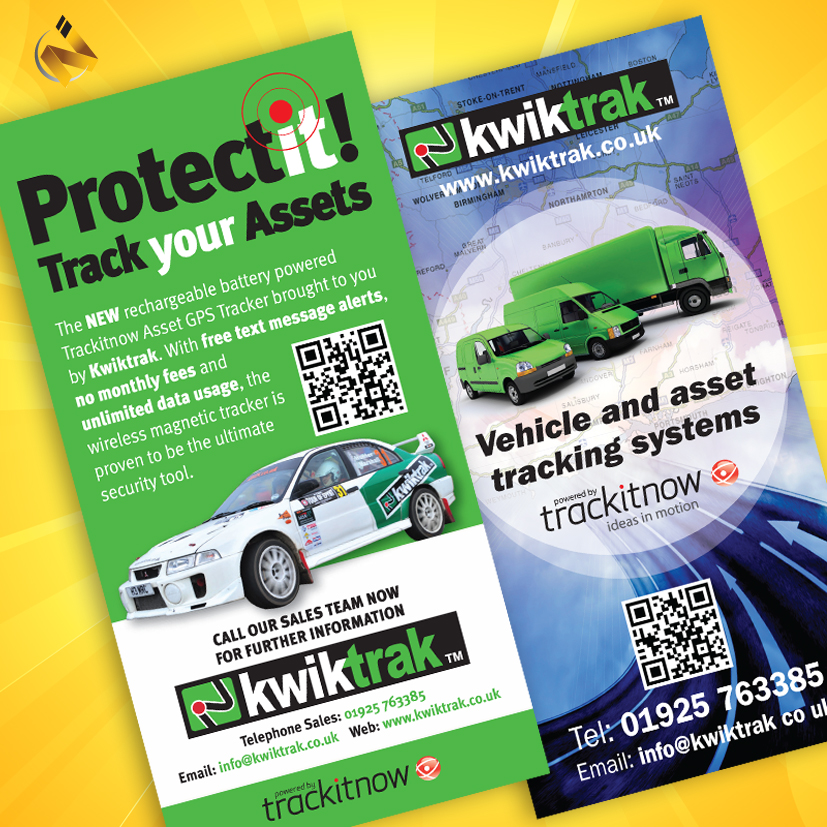The image depicts a promotional brochure for QuickTrack's vehicle and asset tracking system, presented in a vibrant layout with detailed information spread across two sections. The left side, set against a green background, emphasizes the slogan "Protect it! Track Your Assets" and introduces QuickTrack's new rechargeable, battery-powered GPS tracker. This section highlights key features such as free text messaging alerts, no monthly fees, and unlimited data usage. A prominent QR code sits above an image of a white Mitsubishi Evo rally car branded with the QuickTrack logo. The bottom portion provides contact details, including a UK sales number, an email address (info@quicktrack.co.uk), and the company's website (www.quicktrack.co.uk).

The right side is characterized by a blue-to-purple map-themed background, starting with the QuickTrack logo and website URL at the top. Centered on this page are illustrations of three different green vehicles—a small delivery van, a sprinter van, and a lorry—emphasizing the system's versatility. Beneath the vehicles, the text reads "Vehicle and Asset Tracking Systems, Powered by TrackItNow," followed by the tagline "Ideas in Motion" in smaller print. A QR code placed below these elements, along with additional contact details, mirrors the information from the left side, ensuring comprehensive coverage and ease of access for potential customers.